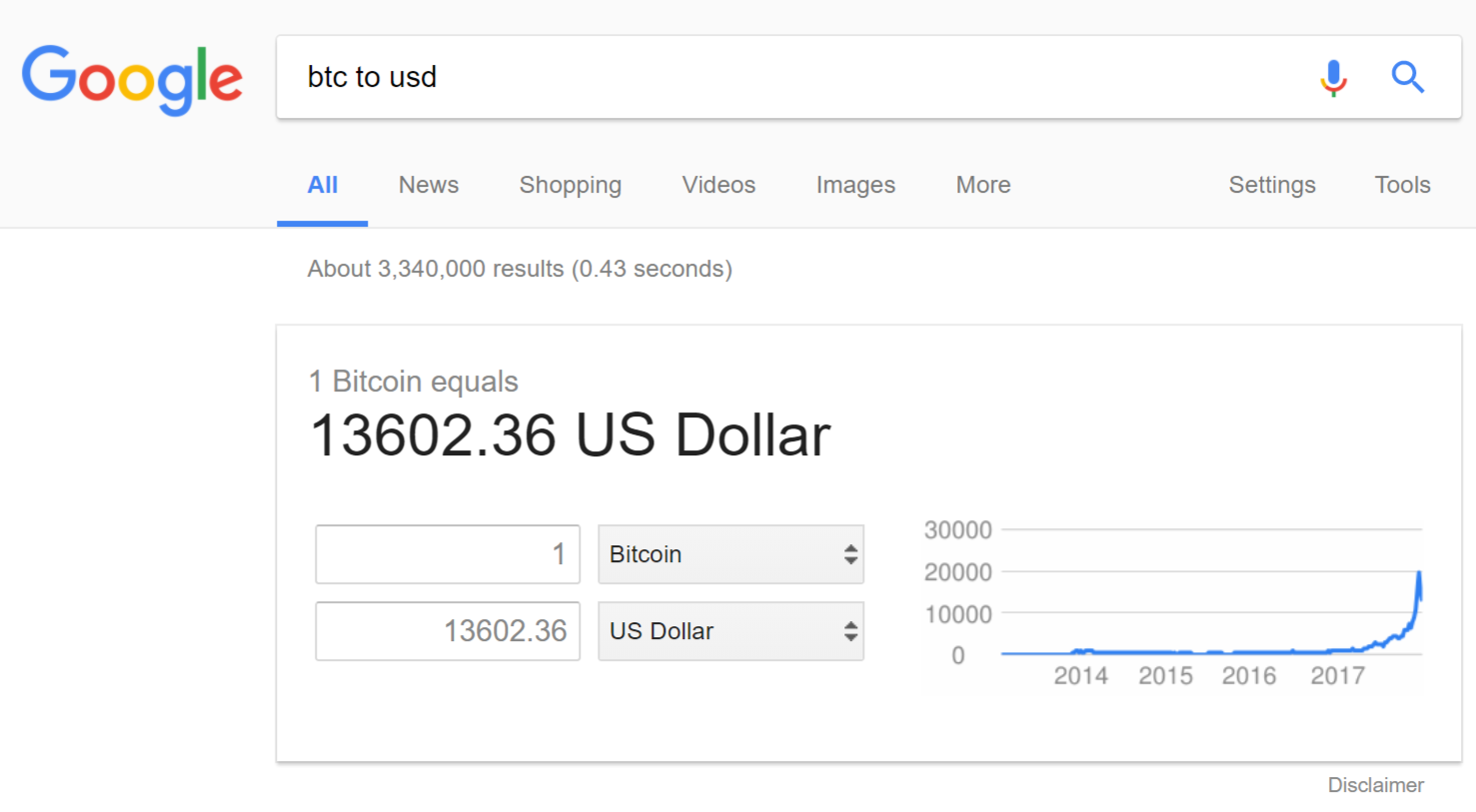A screenshot depicts a Google search page in light mode, displaying the query "BTC to USD" in lowercase letters. The interface features the typical white and blue Google color scheme, with no special or historical designs in the logo. The primary search result is prominently shown in a conversion box, indicating that 1 BTC equals $13,602.36 USD. Adjacent to this, on the right side, is a small chart illustrating the historical conversion rate of Bitcoin (BTC) from 2014 to 2017, highlighting a notable increase in value over this period. The search bar at the top includes a microphone icon and a magnifying glass icon, with tabs for All, News, Shopping, Videos, Images, More, Settings, and Tools available for further navigation.